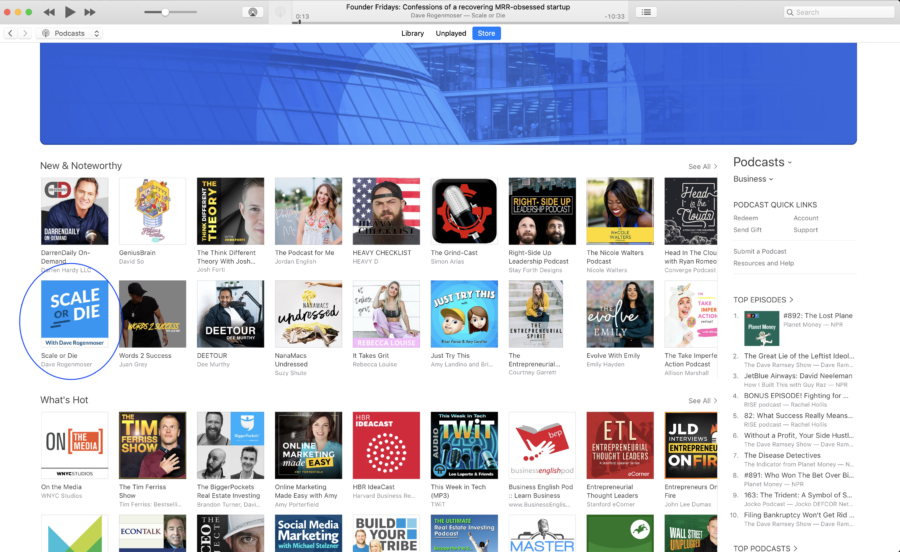This image is a detailed screenshot of a podcast listening app, likely displayed on an Apple computer, showcasing various options and features for the user. Here's a refined and descriptive caption for the image:

---

**Detailed Screenshot of a Podcast App on an Apple Computer**

This screenshot captures a podcast streaming app on an Apple computer. The interface is divided into multiple sections with various functionalities.

### Top Browser Bar:
- **Three Circles (Top Left)**: These classic MacOS window management buttons are colored red, yellow, and green, respectively.
- **Playback Controls (To the Right)**: Includes a "skip left" button, a "play" button, and a "skip right" button.
- **Volume Slider**: Accompanied by an unidentified icon within a light gray rectangle.
- **Title and Playback Information (Centered)**: Displays the title "Founder Fridays: Confessions of a Recovering M.R.R. Obsessed Startup" in bold black letters. Beneath it, in lighter text, the subtitle reads, "Dave ... Scale or Die". A playback progress bar shows the user is 13 seconds into a total duration of 10 minutes and 33 seconds. An additional unfamiliar icon and a search bar are located further to the right.

### Navigation Bar (Below Browser Bar):
- Features navigation buttons for browsing podcasts, including "Library," "Unplayed," and a "Store" button, the latter highlighted with a blue rectangle.

### Main Content:
- **First Row (Heading: "New and Noteworthy")**: Shows thumbnails of various podcasts, with each featuring an image followed by the podcast’s name in text beneath. Examples include an image of a man with the text "Darren Daly On Demand" and more thumbnails featuring recognizable figures like Michelle Obama.
- **Highlighted Podcast**: A user-added blue circle emphasizes a podcast titled "Scale or Die" with white letters on a blue background, and the name "Dave ... Origin Viewer" is visible below it.
- **Subsequent Rows (Heading: "What's Hot")**: Continues to display additional podcast selections in a similar thumbnail format.

### Sidebar (Far Right):
- **Drop Down Menus**: Categories titled "Podcast" and "Business".
- **Quick Links**: Options such as "Redeem," "Account," "Send Gift," "Support," "Submit a Podcast," "Resources," "Help," and a list of "Top Episodes".

### Visuals:
The app interface prominently features a blue-tinted header image resembling a corporate building, enhancing the professional theme.

---

This structured and descriptive breakdown of the screenshot provides a comprehensive view of the podcast app's layout and functionalities, making it easy for a reader to visualize the content and design.